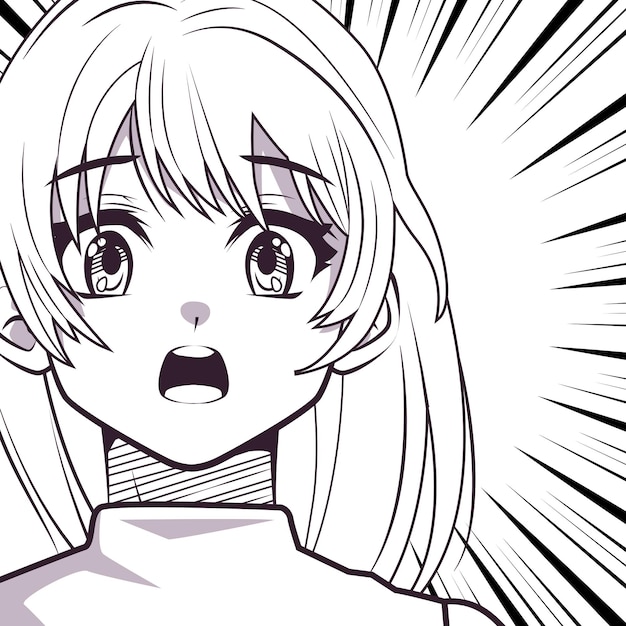This detailed black and white anime-style illustration features a young female character with a Caucasian appearance and long, fair hair highlighted by black lines. Dominating the left side of the image, she has very large, round eyes accented by tears that have yet to fall, giving her an emotional, incredulous expression. Her wide-open mouth reveals white teeth and a blackened inside, and a small, gray button-nose with hints of purple further punctuates her distraught look. Black spikes or sun ray lines emanate from her head, enhancing her shocked demeanor. She wears a white top adorned with subtle purple highlights. The overall grayscale palette is occasionally pierced by these minimal touches of color, emphasizing the character's vivid emotional state.